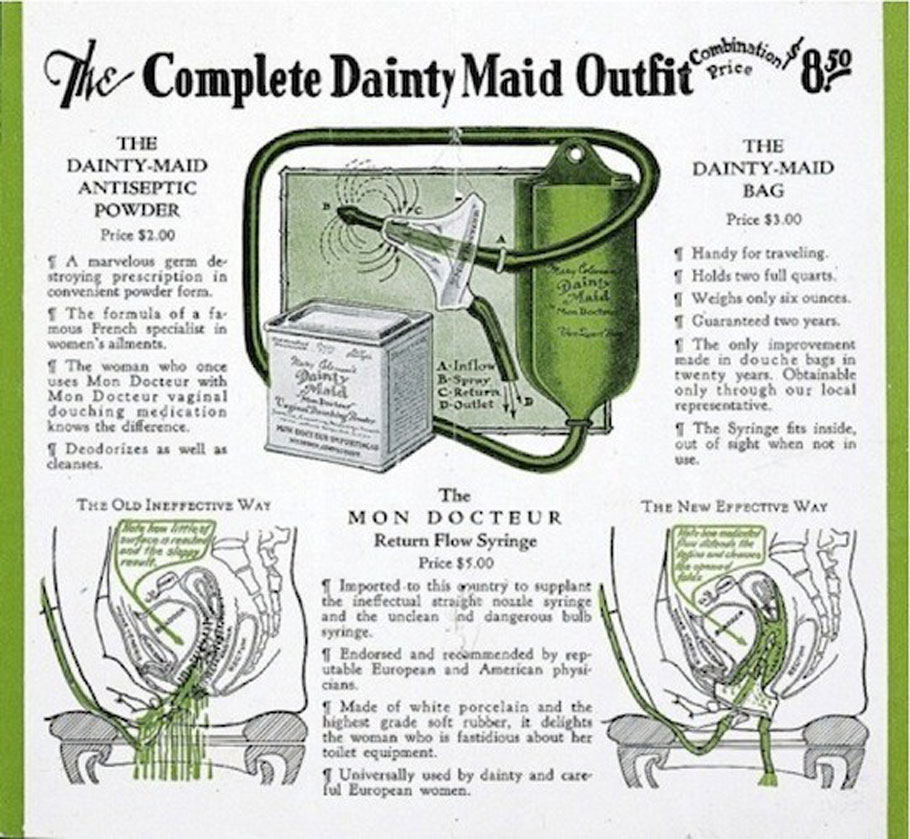This image is an antique advertisement, potentially dating back 100 to 150 years, for "The Complete Dainty Maid Outfit," priced at $8.50. The advertisement showcases a medical device set predominantly in green and white. At the top center, it features the "Dainty Maid Bag," priced at $3, accompanied by the "Dainty Maid Antiseptic Powder," described as a marvelous germ-destroying prescription in powder form, credited to a French specialist in women's ailments.

The Dainty Maid Bag is highlighted as ideal for travel, capable of holding two full quarts while weighing only six ounces, and comes with a two-year guarantee, noted as the only improvement in douchebags in 20 years, available exclusively through local representatives. In the center, there's a depiction of the bag, which resembles an IV bag with a suction cup connected by a green hose.

Below this illustration, another section introduces "The Mondaktor Return Flow Syringe," priced at $5.00, explaining it can be stored out of sight when not in use.

Additionally, the ad juxtaposes two images labeled "Old Ineffective Way" and "New Effective Way," illustrating the device's use, with the newer method indicated to function better, despite both images appearing quite similar. The whole set emphasizes convenience, efficacy, and modern hygienic advancement over traditional methods.